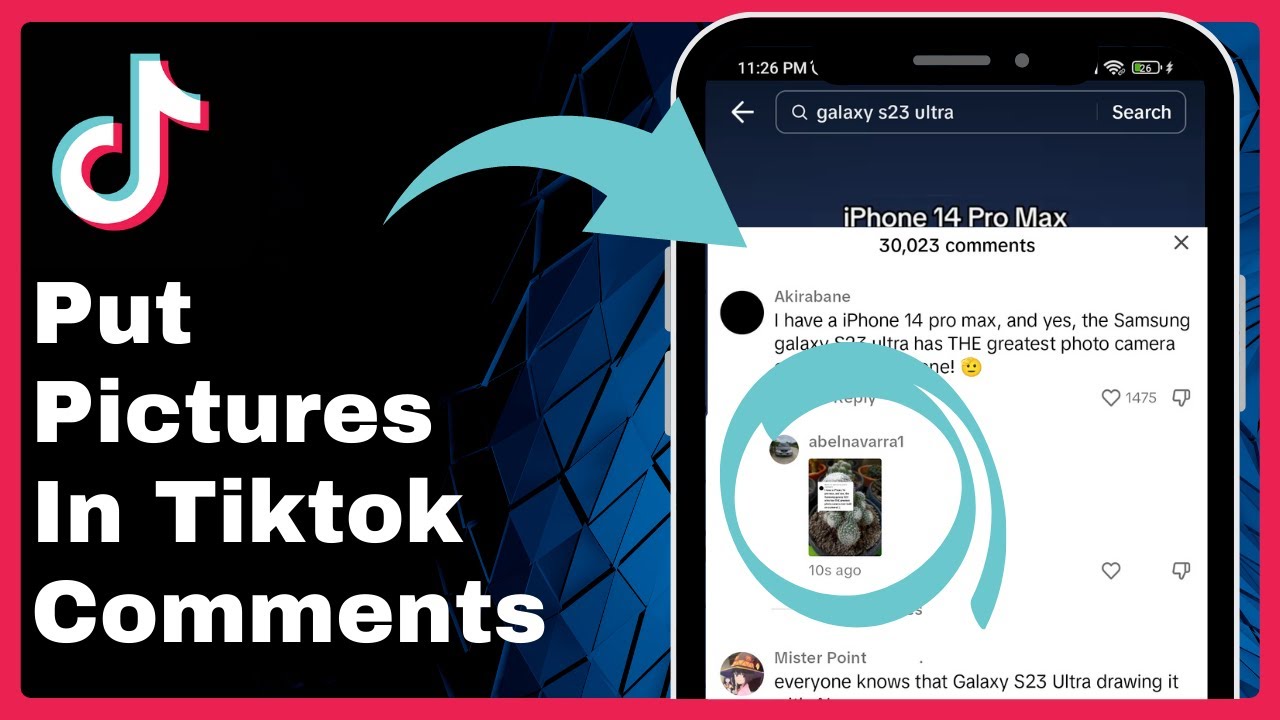Certainly! Here is a cleaned-up and detailed caption for the described image:

---

The image showcases a large, old-style website bordered with red trim, set against a deep navy blue background. On the right side of the page, there is a mock-up of a smartphone displaying the TikTok app interface. The TikTok icon is prominently featured, with instructions on how to add pictures to TikTok comments, illustrated by an aqua-colored arrow. 

The mock-up phone display reads "11:26 PM" with approximately half battery life and shows "Galaxy S23 Ultra" on its search bar, although the mock-up resembles an iPhone 14 Pro Max. The comments section reveals active user discussions, totaling 30,023 comments. One comment mentions having an iPhone 14 Pro Max and acknowledges that despite the Galaxy S23 Ultra's superior camera, there is something indiscernible beneath it. Another comment, encircled in light blue, asserts that everyone is aware of the Galaxy S23 Ultra's high-quality drawings, yet is another entry into the ongoing debate between iPhone 14 and Samsung Galaxy users.

---